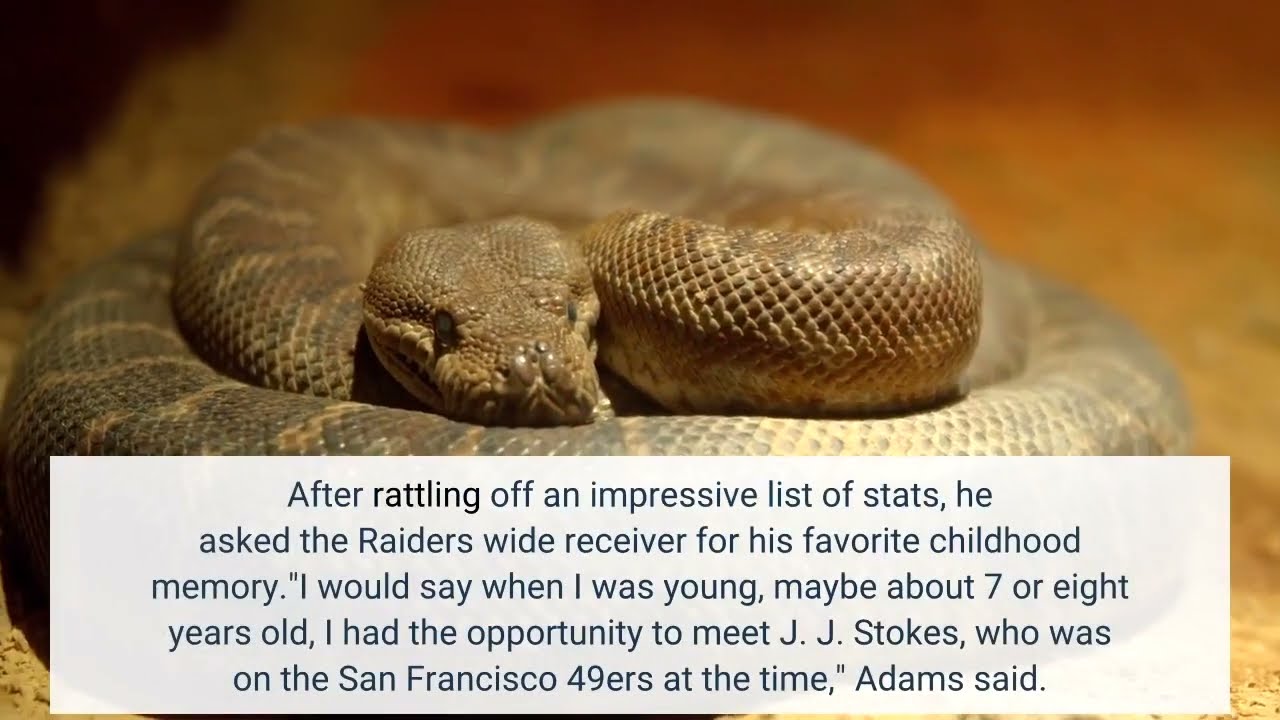The image depicts a coiled brown snake with a mix of gray and intricate dark and light markings, resembling a python. The snake's head faces the viewer, with its alert eyes and snout clearly visible. The background is a blurred, warm blend of orangish tones that creates a stark contrast, accentuating the snake's details. At the bottom of the image, a white rectangular box encases text, narrating a memory where a Raiders wide receiver reminisces about meeting J.J. Stokes of the San Francisco 49ers during his childhood. The text reads: "After rattling off an impressive list of stats, he asked the Raiders wide receiver for his favorite childhood memory. 'I would say when I was young, maybe about seven or eight years old, I had the opportunity to meet J.J. Stokes, who was on the San Francisco 49ers at the time,' Adams said." The white box partially covers one of the snake's coils, blending the narrative with the captivating visual.